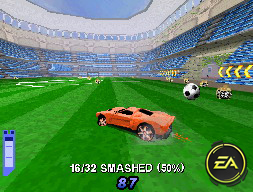The screenshot depicts a classic EA Electronic Arts video game, likely from the late '80s or early '90s, featuring an orange sports car, potentially controlled by the player. The car is driving across a green, grass-like soccer field within an unusually large, empty stadium with animated blue seats. Above the back of the car, an oversized soccer ball is seen bouncing, suggesting gameplay similar to the modern "Rocket League." In the middle left of the screen, game stats are displayed: "16 / 32 smashed, 50%" and a score of "87." The bottom right corner of the screen prominently features the EA logo, styled in black and yellow. The sky above is visible, indicating an open-top stadium design, which, together with the pixelated graphics, reflects the game’s vintage origin.